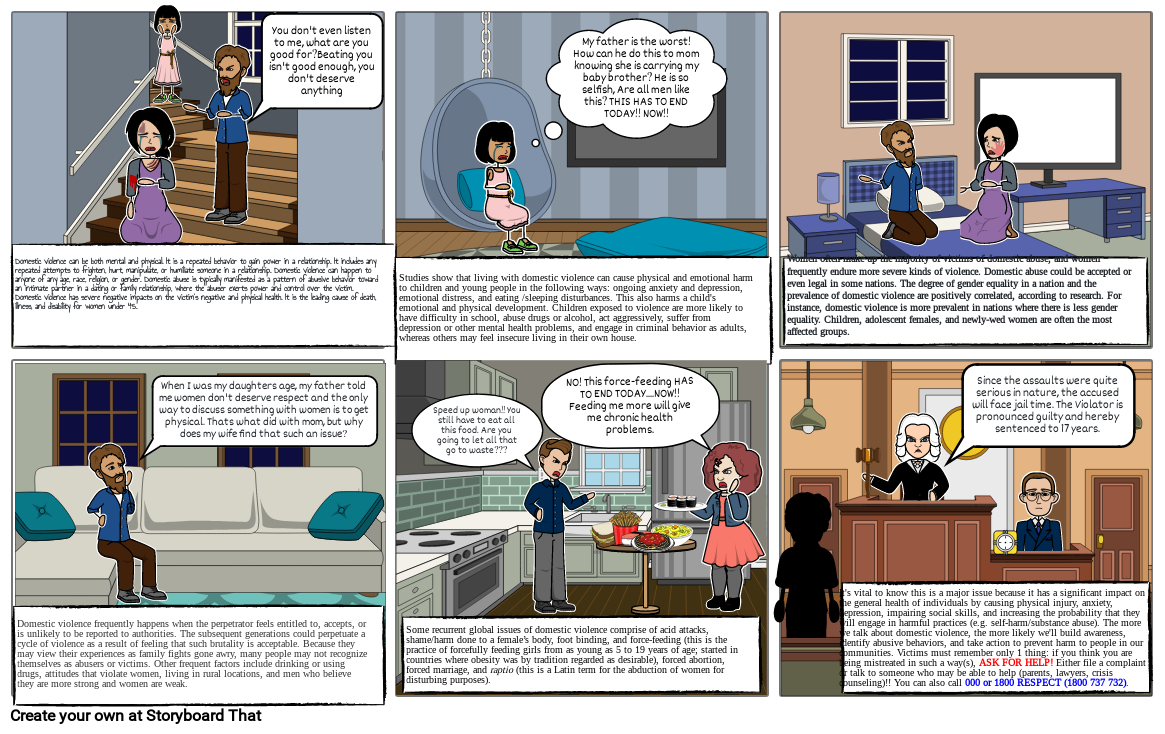This colorful six-panel cartoon strip is arranged in two rows, each containing three panels. In the first panel, a family of three—a man, a woman, and a child—are standing on a staircase with blue walls. The man, with brown hair, a blue shirt, and brown pants, is midway down the stairs, gesturing with his palms facing upward while speaking. Behind him is a young girl in a pink dress with black hair, and at the bottom of the stairs stands the woman in a purple dress with gray sleeves, appearing distressed.

In the second panel, the young girl is seated in an egg-shaped light blue chair with a blue throw pillow, suspended from a silver chain in a room with blue-striped walls. She seems to be lost in thought, with a thought balloon above her. The third panel shows the man and woman kneeling on a bed, seemingly engaged in conversation.

The fourth panel transitions to the man alone, now sitting on a tan couch with a blue throw pillow at each end, continuing to speak. In the fifth panel, a different scene unfolds in a kitchen where the man is seen with another woman in an orange dress, possibly arguing. The final panel presents a courtroom scene with a judge poised to strike the gavel, a silhouette of a figure standing before the judge, and a court clerk positioned to the judge's left. The dialogue throughout the strip is unreadable, adding an element of mystery to the narrative.